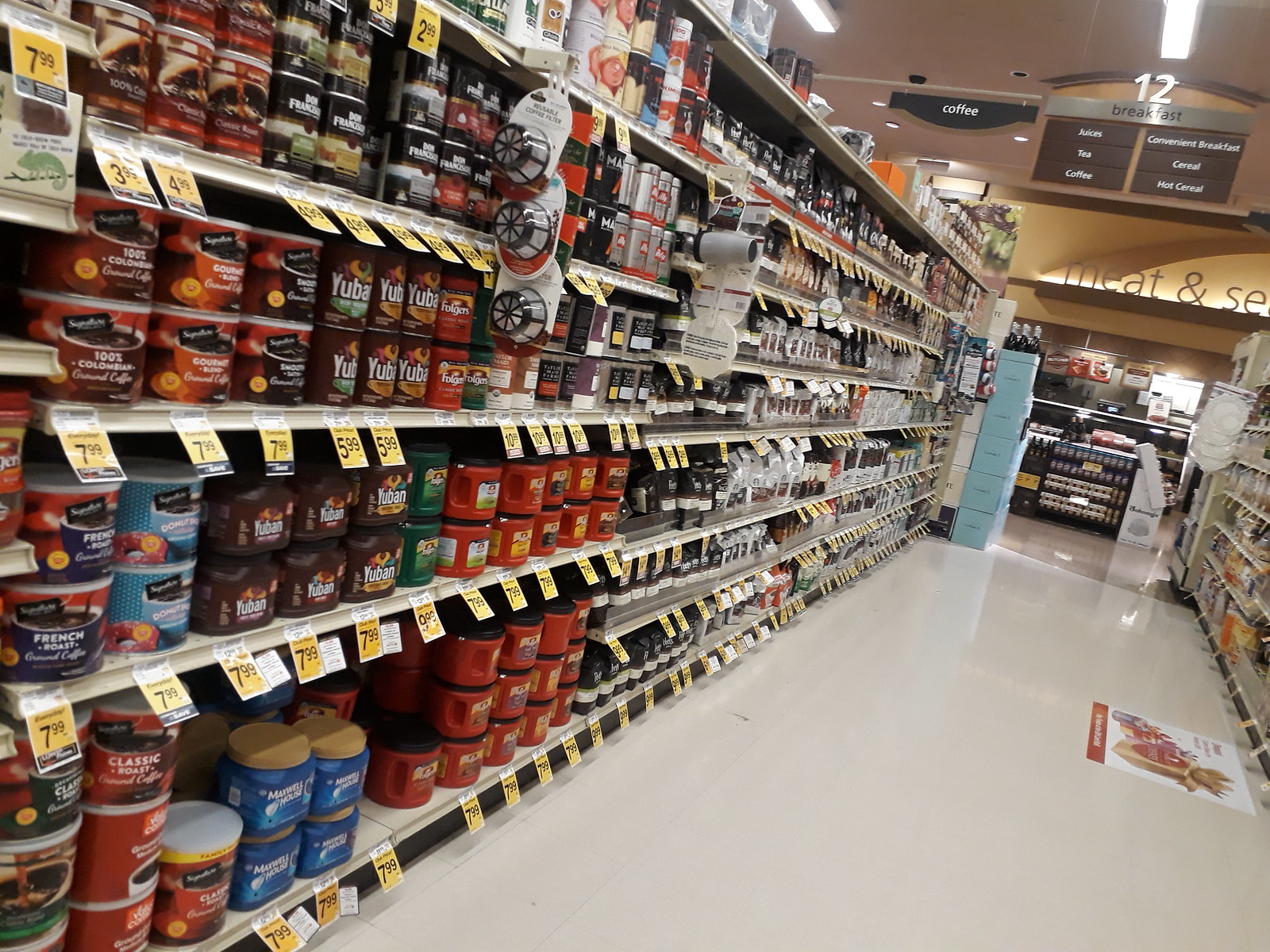A meticulously organized aisle in a bustling grocery store is captured in this image. The pristine white floor contrasts with the densely packed shelves that flank both sides of the aisle. At the top of the image, a sign indicating "Breakfast 12" informs shoppers that they are in the breakfast section, which houses a variety of products including tea, coffee, and cereal.

To the immediate left, a diverse assortment of coffee brands is prominently displayed, with notable labels such as Yuba and a French Roast variety in medium-sized, canned containers. Suspended from the upper shelves are various coffee-related accessories, including what appear to be coffee filters or drip devices, essential for any coffee aficionado. Further down the left side of the aisle, a selection of stylish coffee tumblers can be seen hanging, ready to cater to customers on the go.

As the eye travels towards the end of the aisle, bottles containing what seems to be sauces are visible, suggesting a transition into another section of the store. The photograph not only showcases the wide variety of breakfast items available but also highlights the meticulous arrangement that makes for an efficient and pleasant shopping experience.